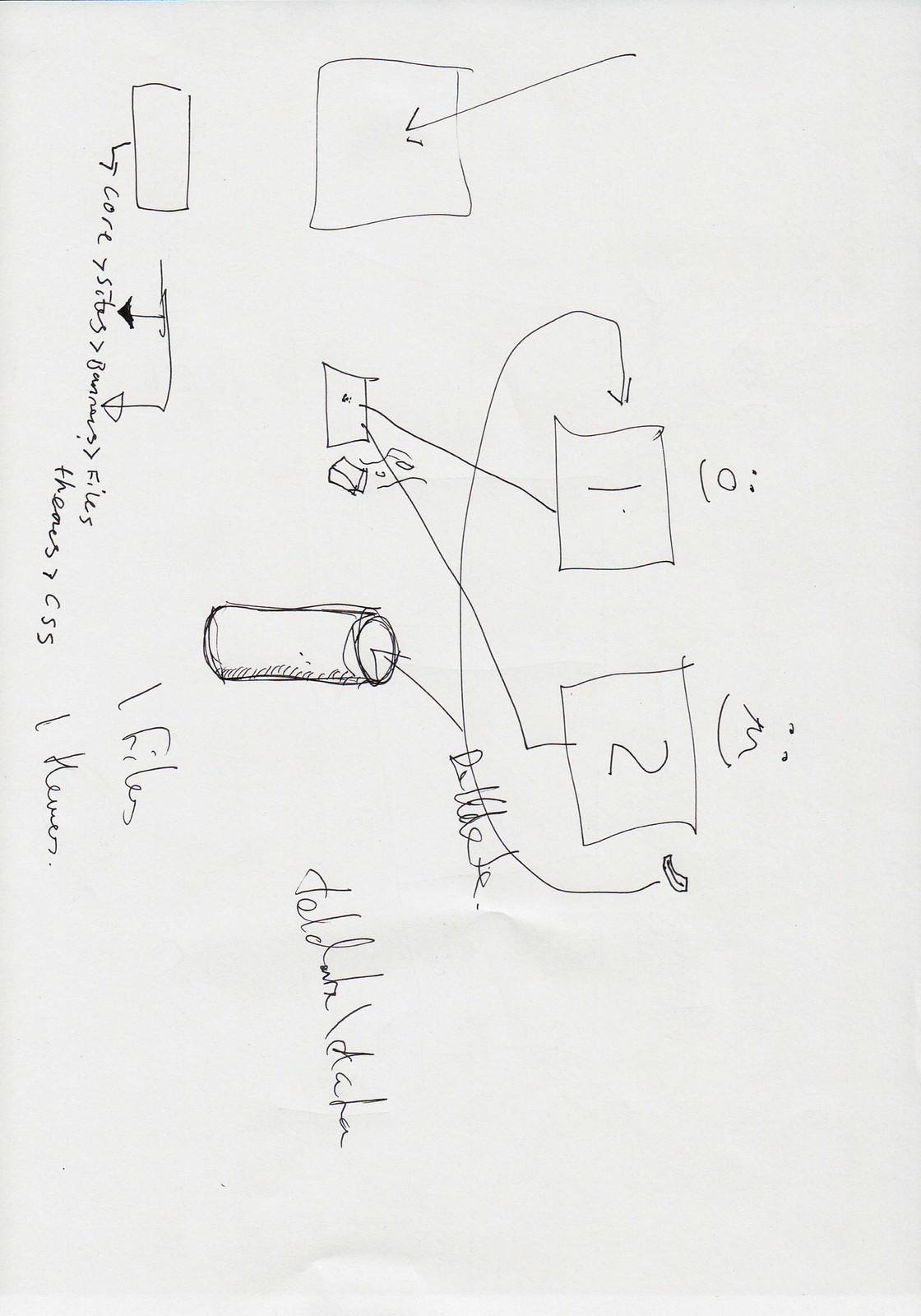This detailed black ink drawing on a white sheet of paper appears to represent a basic network flowchart. Though intended to be viewed in landscape orientation, the description provides a portrait view framework:

- At the top, there are two distinct face-like structures. The first one consists of two dots for eyes, a circle for a nose, and a semi-smiley face representing a mouth. The second one, to the right, features two dots above an 'M' shape reminiscent of a nose, coupled with a smiley face.
- Beneath each face are two squares. The square on the left contains the number "1," while the square on the right contains the number "2."
- Connecting these squares are lines that lead to additional boxes. 
- Some arrows extend from each box's side, directing downwards to a container.
- Underneath this container, the text, written in messy cursive, reads, "one files, a can," and another indiscernible phrase.
- On the left side of the drawing, an additional box is marked with an arrow pointing towards it.
- Below this box, there's a rectangular shape featuring a small arrow pointing to it, with the label "core" followed by an illegible cursive word, "files," and the term "CSS."

This diagram, likely sketched by a network administrator or engineer, illustrates a rudimentary flowchart outlining a network’s structure or data flow, with various elements such as nodes, containers, and core files referenced.